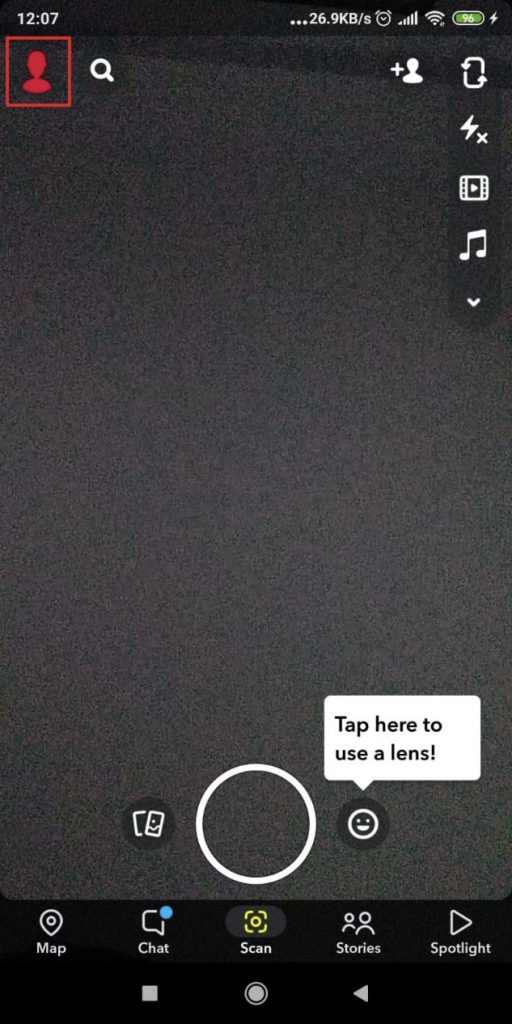In the top left corner of the image, there is a silhouette of a person marked in red next to the number "1207," along with a Wi-Fi symbol and an alarm icon. Underneath, a battery icon is visible, alongside a search button. The image also includes a second silhouette of a person with an arrow pointing towards them. Two arrows form a circular pattern, symbolizing rotation or refresh, and a lightning bolt with a crossed-out mark indicates a prohibition of some electrical function. Additionally, movie and film reel icons, a music note symbol, and an arrow are present. At the bottom center of the image is a large circle flanked by two smaller pictures, followed by another circle. The text "Tap here to use a lens" appears prominently. Lower down, there are navigation options labeled "Map," "Chat," "You," "Friends," and "Spotlight." The bottom right features a square, a circle, and another arrow.